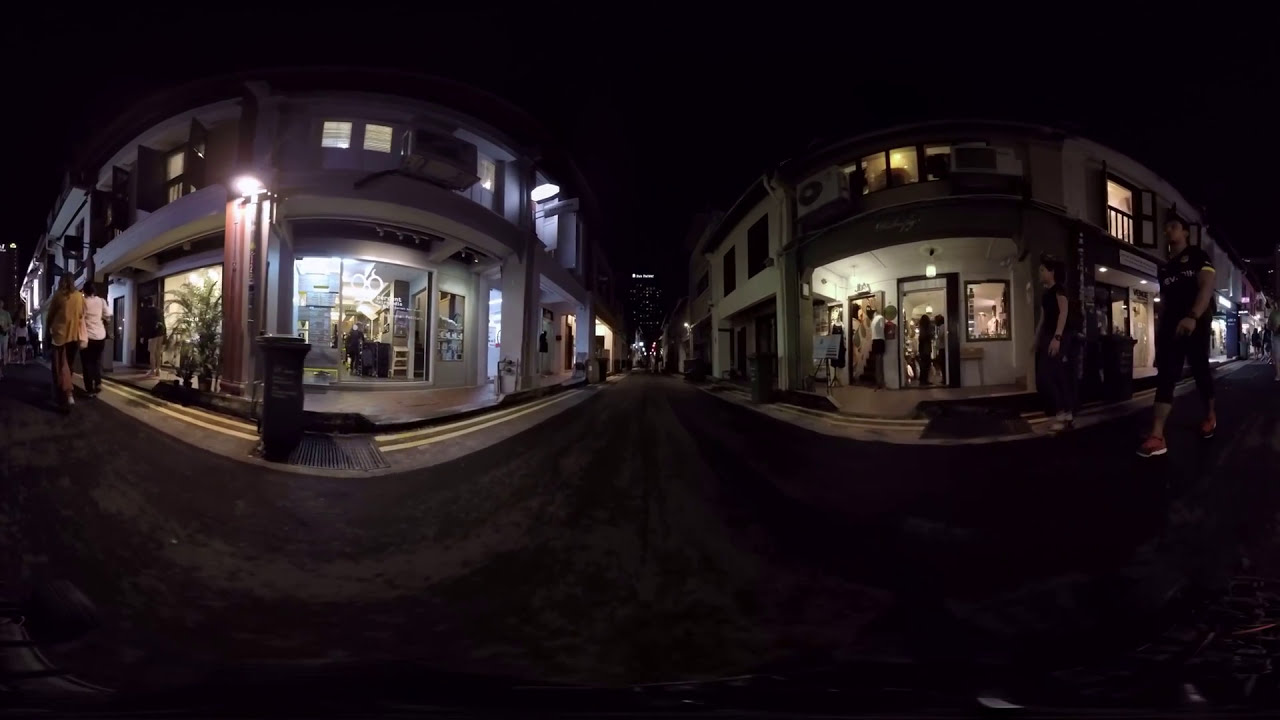A nighttime photograph of a city intersection captures a fisheye effect, making the scene appear curved. On either side of the dark grey road, two buildings stand prominently, their white walls illuminated by streetlights. The building on the right is rounded, bustling with people entering and exiting, and features a trash bin and few plants near its entrance. This building also has apartments on the upper floors. The left-hand building, which appears to have large plate glass windows, looks like a storefront currently closed, with an air conditioner and window shutters visible on the second floor. The street is alive with pedestrians: people walking along the streets on both sides and additional individuals near the right building's doorway, possibly indicating a restaurant. The sky above is pitch black, emphasizing the lit sign at the far end of the road, which remains unreadable from this distance.